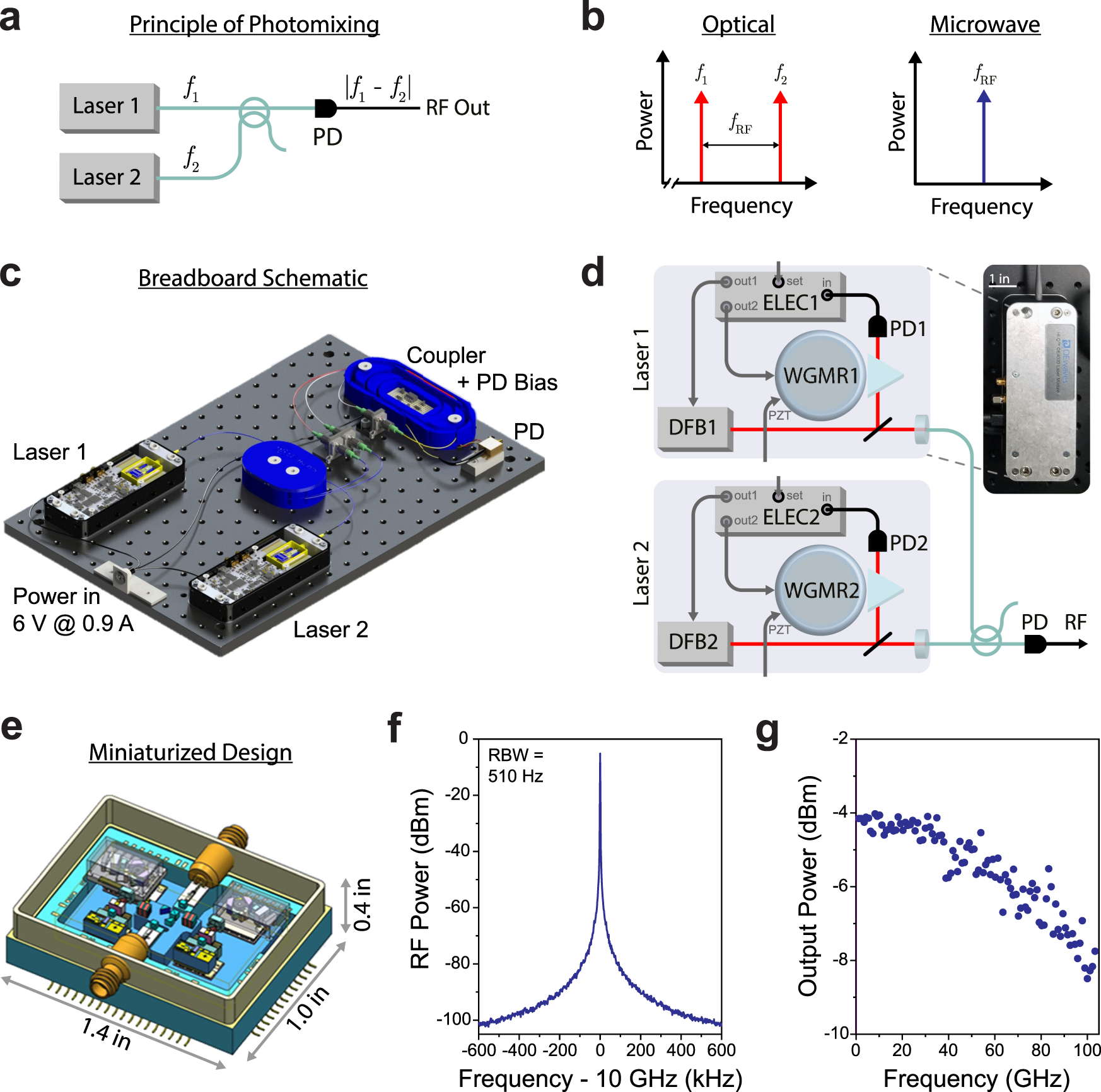The infographic comprehensively illustrates the principle and design of an electronic device, segmented into sections labeled A through G. 

- **Section A** explains the "Principle of Photomixing" featuring a diagram with two lasers (laser 1 and laser 2) and their corresponding formulaic equation.
- **Section B** presents two mini-graphs labeled "optical" and "microwave," both depicting frequency on the Y-axis.
- **Section C** details "Breadboard Schematics," showing a layout including laser 1, laser 2, a blue coupler, and PD bias on a gray rectangular base, with gears depicted as blue elements. The lasers are represented as black rectangular boxes.
- **Section D** provides a close-up schematic for laser 1 and laser 2, highlighting where the electricity is routed and additional specifications for each laser.
- **Section E** shows a "Miniaturized Design" of a laser.
- **Section F** includes a graph where the Y-axis is labeled RF power, and the X-axis represents frequency with increments in gigahertz or kilohertz, displaying a line graph with values ranging from negative 100 to nearly zero.
- **Section G** features another graph labeled "Output Power (dBm)" on the Y-axis and "Frequency (GHz)" on the X-axis, with a dotted line moving from negative 4 on the almost top right to 130 on the bottom left.

Overall, the infographic combines diagrams, schematics, and frequency graphs to illustrate the design and function of an electronic device involving photomixing and lasers.